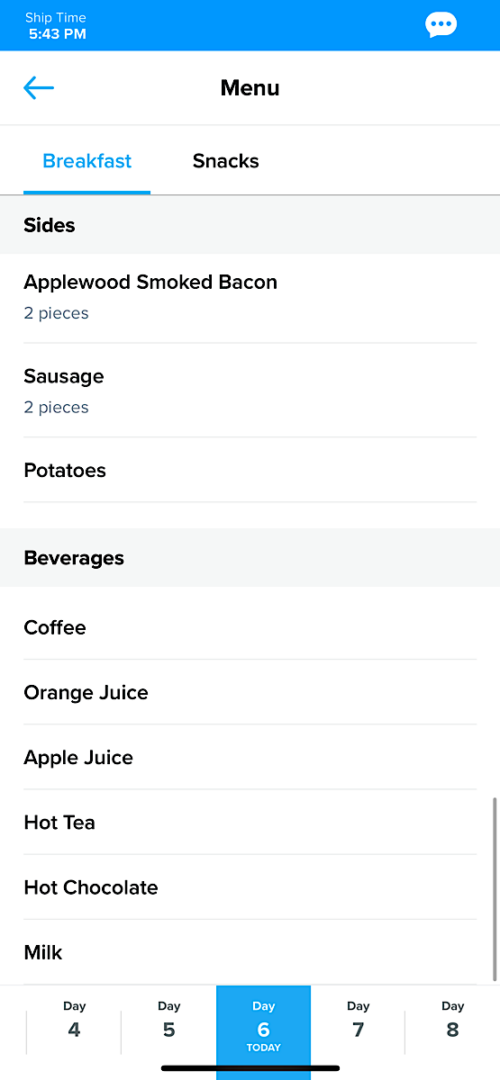The image displays a menu screen with various details. In the top left corner, it indicates the current time as "Ship Time: 5:43 PM." The top right corner features a blue chat bubble icon, a back arrow, and a menu button, all in blue. The main heading "Breakfast" is shown with a blue underline, and "Snacks" is listed in black to its right. The breakfast menu includes items such as Applewood smoked bacon (two pieces), sausage (two pieces), potatoes, and a selection of beverages including coffee, orange juice, apple juice, hot tea, hot chocolate, and milk. Below this section, there is a date navigation bar with days labeled as "Day Four," "Day Five," "Day Six" (highlighted in blue as today), "Day Seven," and "Day Eight." The bottom of the screen has a black line, the right side features a gray line, and the image has a blue border at the top.